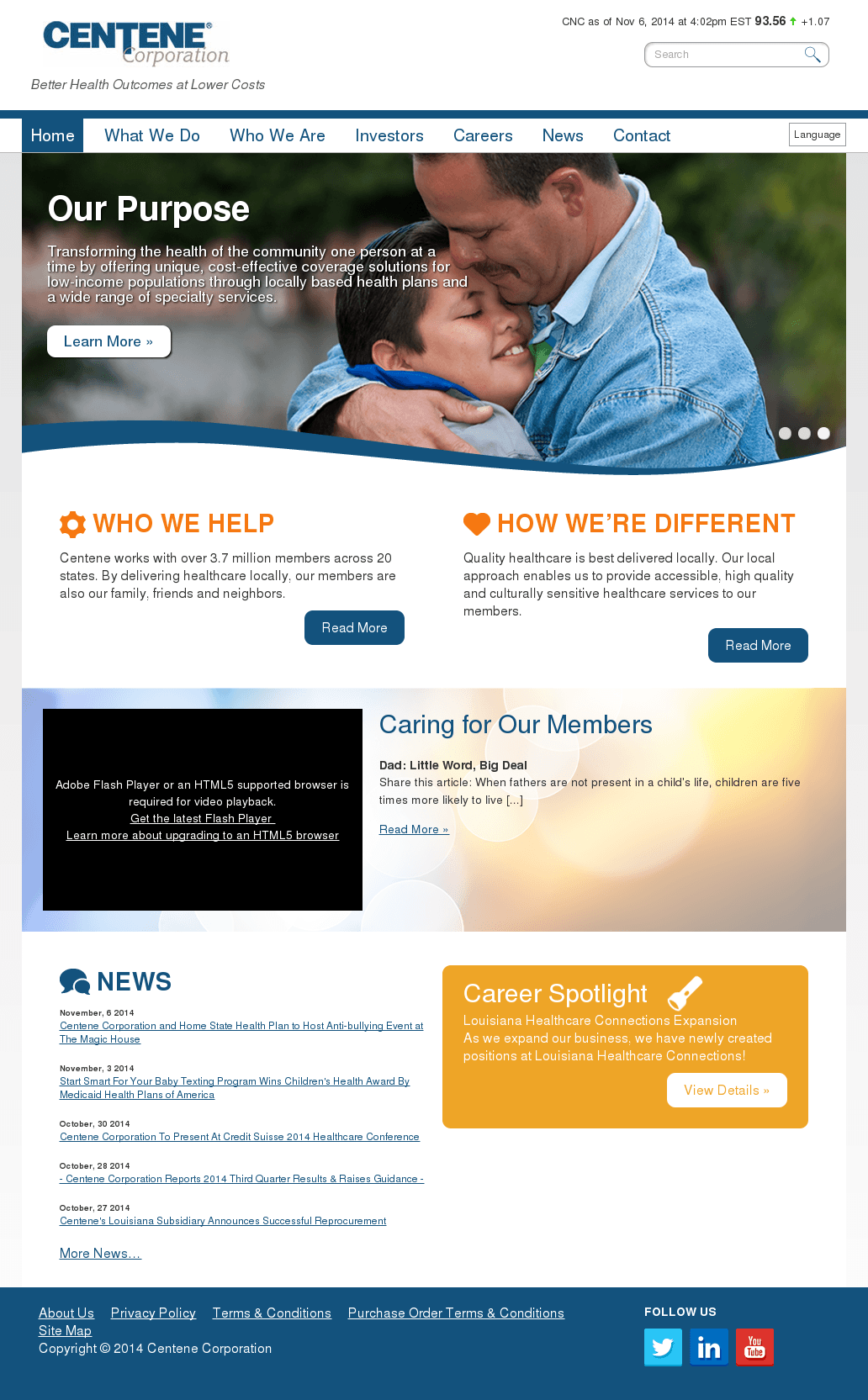This is a detailed screenshot capturing the homepage of Centene's website. The company name, "CENTENE," is prominently displayed in all capital letters in dark blue text positioned on the top left corner against a white background. The top border features a navigation menu, highlighted at the very top by a thin dark blue line. The menu itself is predominantly white, with the first item, "Home," displayed in white text within a dark blue box. The subsequent menu items are in dark blue text within white boxes and include: "What We Do," "Who We Are," "Investors," "Careers," "News," and "Contact."

On the top right corner, there is a search box for user convenience. Just below the menu, the main header reads "Our Purpose" in large, bold text, accompanied by smaller white text that provides further details. Centered on the page is a heartwarming image of a man embracing a young boy. Adjacent to the image is a white call-to-action box that says "Learn More."

The section below the header and image is divided into multiple text boxes of varying colors, including white, dark blue, and orange. Each box has a distinct header, such as "Who We Help," "How We Are Different," "Caring for Our Members," "News," and "Career Spotlight."

At the very bottom of the page, a dark blue banner spans across, containing small white text. In the bottom right corner of this banner are icons linking to Centene's social media platforms: Twitter, LinkedIn, and another platform denoted by a red box.